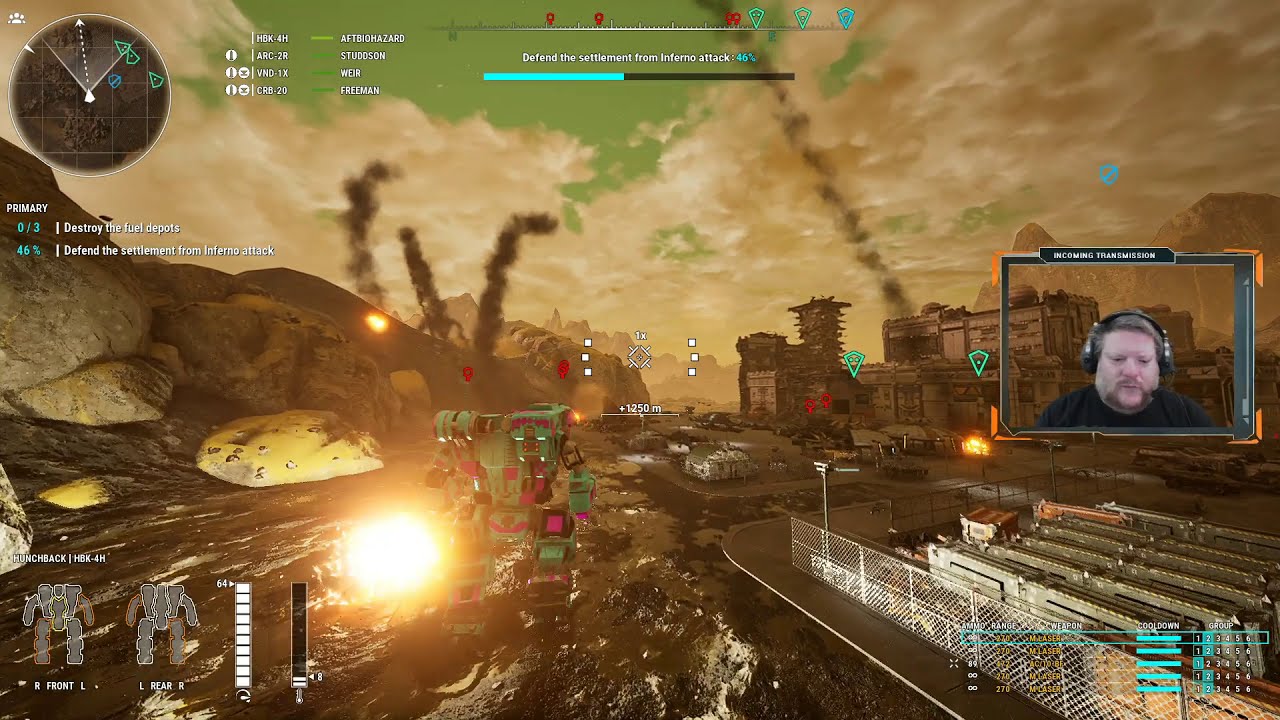In this detailed scene taken from a video game, we observe a complex and war-torn environment. The image predominantly features shades of brown and olive, highlighted by rising smoke and scattered explosions. A significant visual element is a large, headless robot, colored in shades of green with purple splotches, moving through what appears to be a partially destroyed industrial town, perhaps a factory area. Behind a chain-link fence lies an electrical grid, adding to the dystopian atmosphere. Above, brown clouds fill the sky, with hints of green and olive smoke, creating a chaotic and eerie ambiance. The ground appears to be covered in tar-like substance, furthering the grim setting.

In a smaller window within the image, situated on the right side, a gamer with brown hair, a goatee, and a black shirt can be seen. He is equipped with a headset and is actively streaming his gameplay. Various scores and measurements are displayed at the top of the screen, indicating the players' progress, suggesting they are about a third to halfway through the game. The presence of bombs can be observed mid-flight, intensifying the sense of active conflict. The scene includes symbols on the damaged buildings, which might denote shooter elements, and hints at a bleacher-like area surrounded by a fence, where four players might be participating in the game.